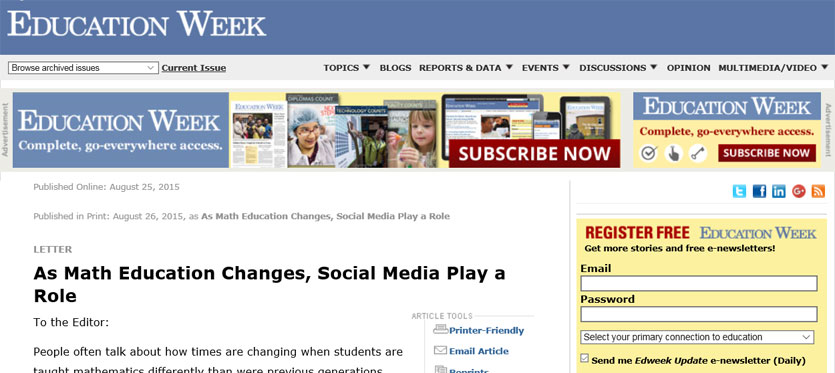This image showcases the homepage of the "Education Week" website. The header features the "Education Week" logo prominently on both the top-left and top-right corners, set against a blue background. Below the header is a navigation bar with tabs labeled 'Browse Archived Issues,' 'Current Issue,' 'Topics,' 'Blogs,' 'Reports & Data,' 'Events,' 'Discussions,' 'Opinion,' and 'Multimedia/Videos.'

In the left sidebar, an advertisement for "Education Week Complete" offers extensive access to all their content, also set against a blue background. Behind this text, there is a faint image of stacked books. A red button labeled "Subscribe Now" is prominently placed below this message.

On the right side, another section repeats the "Education Week Complete" offer on a blue background, but the accompanying text "Go Everywhere Access" is highlighted on a yellow background with red text. This section also features a red "Subscribe Now" button.

At the bottom left, it includes publication details: "Published Online: August 25, 2015" and "Published in Print: August 26, 2015," alongside a snippet of an article discussing the changing role of social media in medical education. It mentions how educational methods, especially in subjects like mathematics, are evolving.

On the bottom right, there is a registration form that invites users to register for free access to more content and newsletters. The form fields include spaces for 'Name,' 'Email,' 'Password,' and a dropdown menu to select the user's primary connection to education. There is also a checkbox option to receive weekly updates.

Overall, the page integrates various elements like subscription options, publication information, and user registration, giving it a comprehensive and detailed structure for readers and potential subscribers.